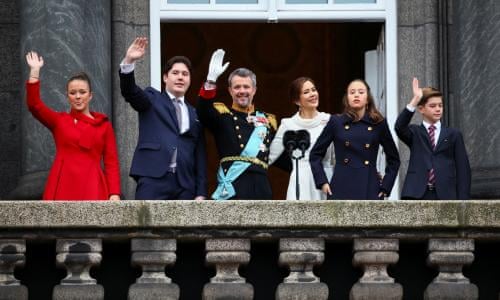This color photograph, likely taken in Europe, showcases a first family of European descent standing on a stone balcony with columns, waving to the public during the daytime. From left to right, there is a woman in a red coat, raising her left hand. Next to her stands a man in a dark suit with a tie, also waving with his left hand. The central figure is a distinguished military officer, approximately in his fifties, adorned with brass buttons, a blue sash, and white gloves, and he too waves with his left hand. To his right, a woman in a formal white dress stands, not waving but smiling warmly. Beside her, a young girl in a navy blue double-breasted peacoat with gold buttons stands with her hands at her sides. Lastly, a young boy, seemingly around 13 years old and dressed in a blue suit, raises his left hand to wave. Mounted together in front of them are two large black microphones, framing the scene as they engage with the onlookers below.